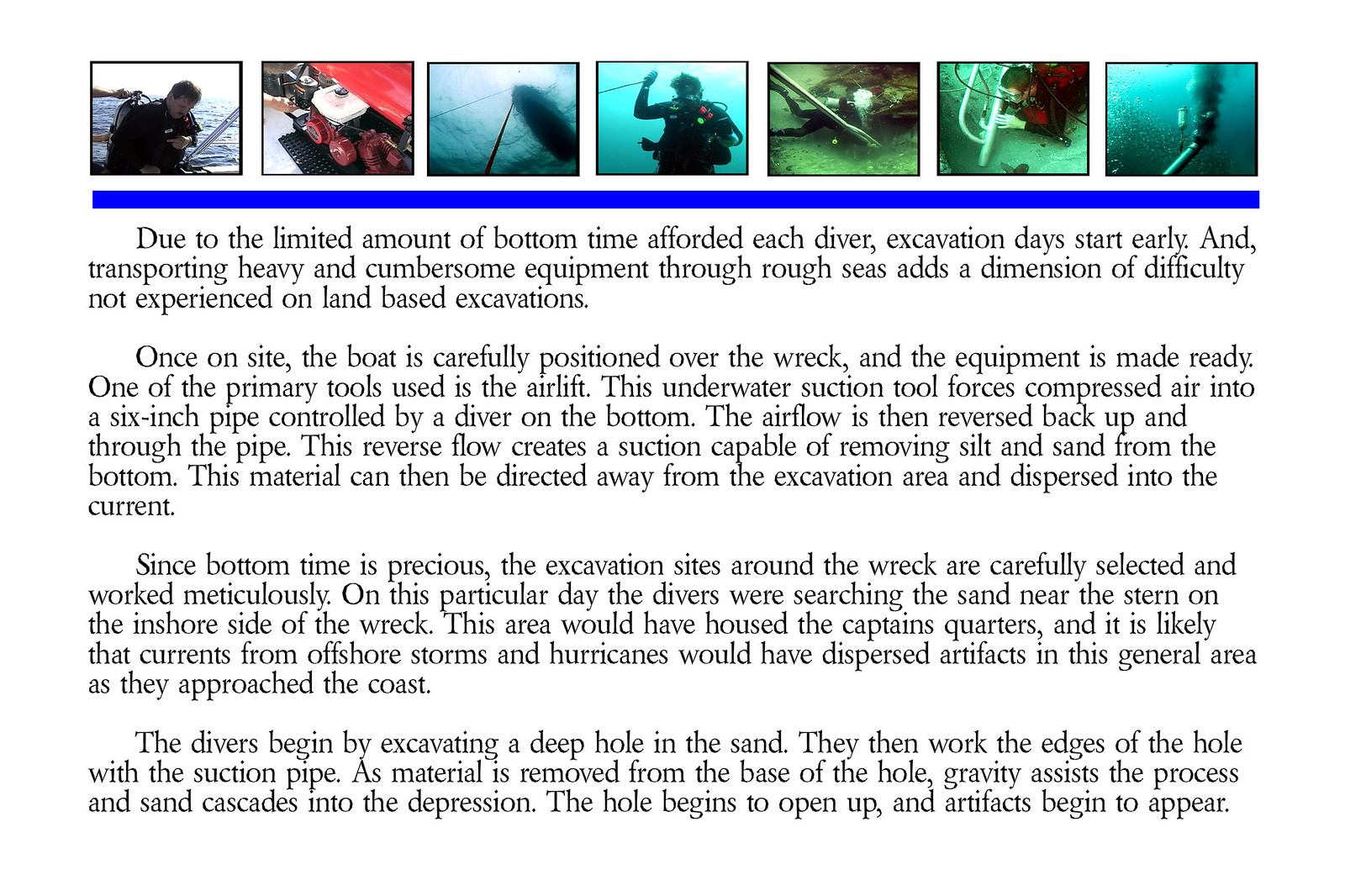This image is a screenshot of an article detailing the arduous process undertaken by a diving team to explore an old shipwreck. The top section features a row of seven small, rectangular photographs, each capturing various stages of the dive setup and exploration: from a diver getting into his wetsuit on the boat, equipment on board, an underwater view looking up at the boat with a rope extended into the water, to divers submerged in the ocean wearing scuba gear. Below these photographs is a horizontal blue bar, which visually separates the images from the textual content beneath. The article itself comprises four paragraphs of black text set against a white background, beginning with a detailed description of the challenges faced by the team, such as the limited bottom time available to each diver and the difficulty of transporting cumbersome equipment through rough seas. It explains the careful positioning of the boat over the wreck and the use of specialized tools like the airlift, an underwater suction tool that injects compressed air into a six-inch pipe, operated by a diver on the ocean floor. The combination of descriptive text and illustrative photographs provides a comprehensive overview of the complex and demanding nature of underwater archaeological excavations.